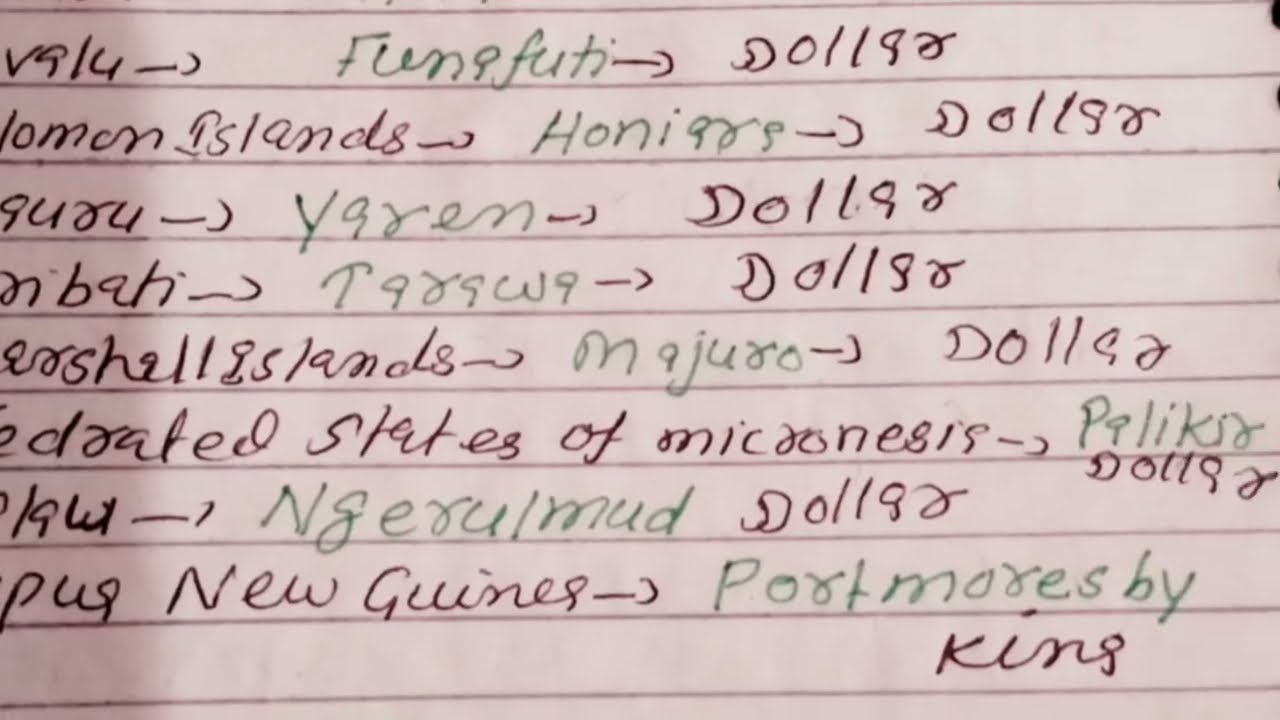The image is a detailed photograph of a lightly colored notebook page filled with handwritten notes in both black and green ink. The page contains various lines and entries, indicating detailed annotations likely related to different geographic locations and currencies. Prominent among the notes are repeated mentions of "dollars" and different islands including "New Guinea," "Solomon Islands," "Micronesian States," and "Marshall Islands." Specific words and names such as "Fanafi," "Dallas," "Guru," and "Palika" appear in varying handwriting and ink colors. Additionally, other less clear terms like "Vo Mon Islands," "Negamon," "Yarin," "Honiarse," and "Postmores by Kings" are noted. The detailed and varied script suggests this could be a travel director's notes from a historical context. All text and objects are upright on the page.